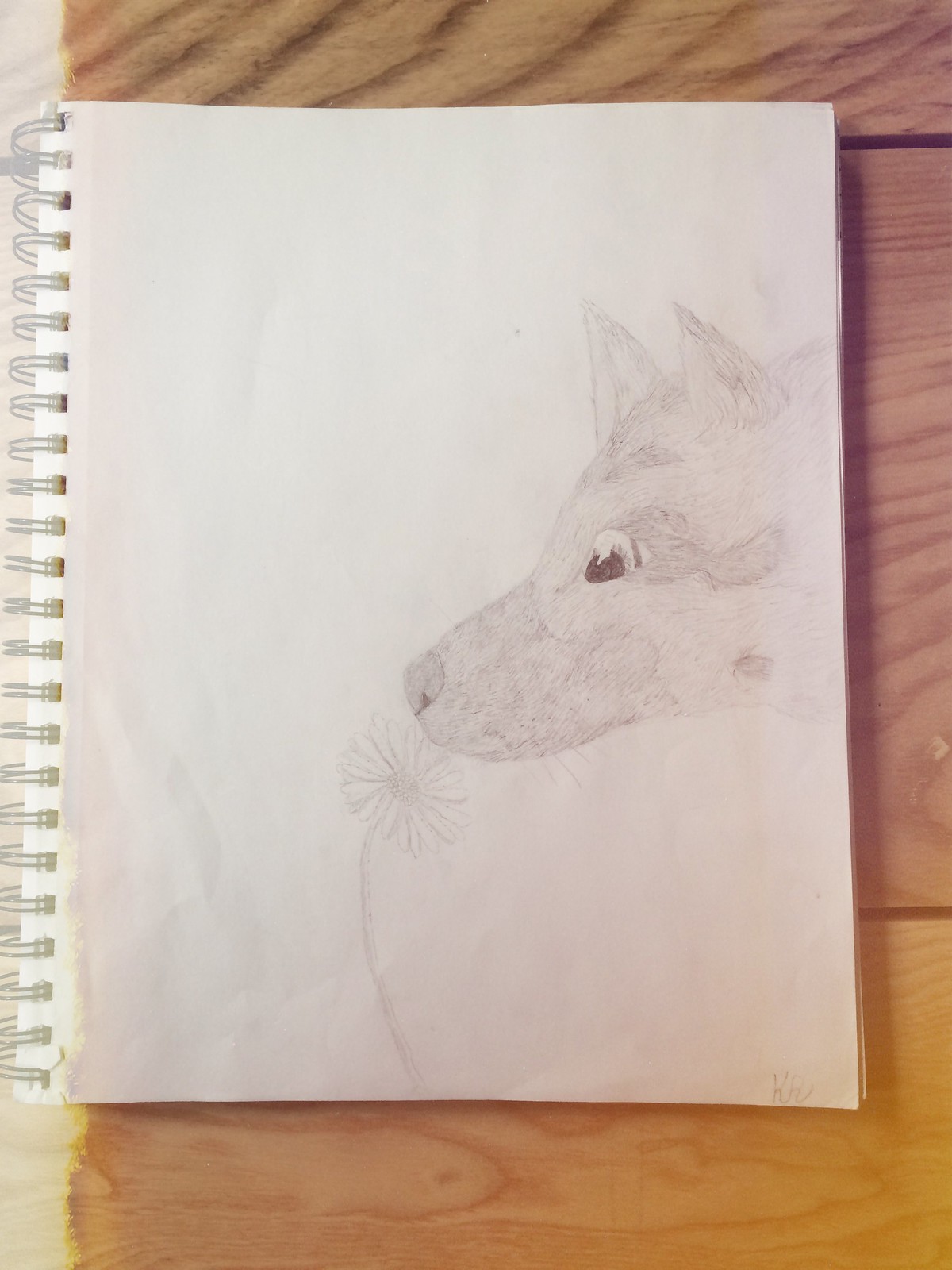The image depicts an open spiral notebook lying on a light wood or light green wood desk. The notebook's pages, which are free of lines, display a pencil sketch of a dog. The sketch captures the dog in a side profile, facing left with intricate details: a dark-colored snout, a light-colored face, and distinctive spots behind the eye and under the chin. The dog's posture suggests it is bending down to sniff a flower on the ground, which appears to be a dandelion. The dog's eye is rendered in white, seemingly illuminated by light. The left edge of the paper in the notebook appears crinkled, and the notebook is bound with white rings on the left, featuring square holes for the rings.